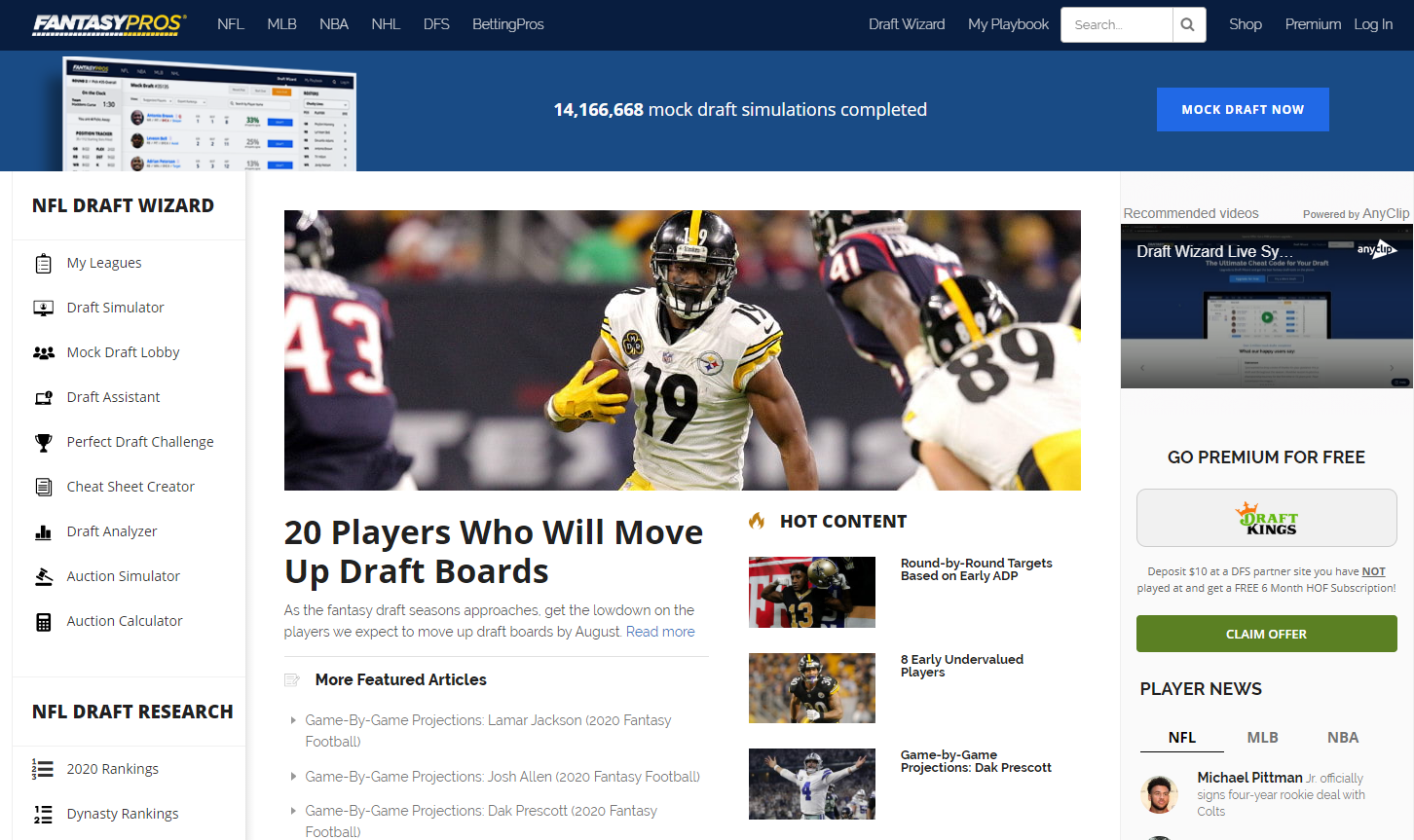The image displays a section of the FantasyPros website, dedicated to sports-related content, potentially including betting. In the upper left corner, the FantasyPros logo is prominently displayed, and the navigation bar spans the top of the page. This bar contains links to various sections including NFL, MLB, NBA, NHL, DFS, and BettingPros. To the right, you can find options labeled "Draft Wizard," "My Playbook," a search bar with a magnifying glass icon, "Shop," "Premium," and "Log In." This navigation bar is styled in a dark blue, almost black strip.

Below the navigation bar, a royal blue section highlights key website features. Prominently showcased in the center is an impressive statistic: "14,166,668 Mock Draft Simulations Completed." Accompanying this is a large, white-font button labeled "Mock Draft Now."

To the left of this central feature, a detailed menu lists various tools and resources, including "NFL Draft Wizard," "My Leagues," "Draft Simulator," "Mock Draft Lobby," "Draft Assistant," "Perfect Draft Challenge," "Cheatsheet Creator," "Draft Analyzer," "Auction Simulator," and "Auction Calculator."

Below these tools is another section dedicated to "NFL Draft Research" with links to "2020 Rankings" and "Dynasty Rankings."

In the middle of the page, there is a prominent image of football players in action, captioned with the text "20 Players Who Will Move Up Draft Boards."